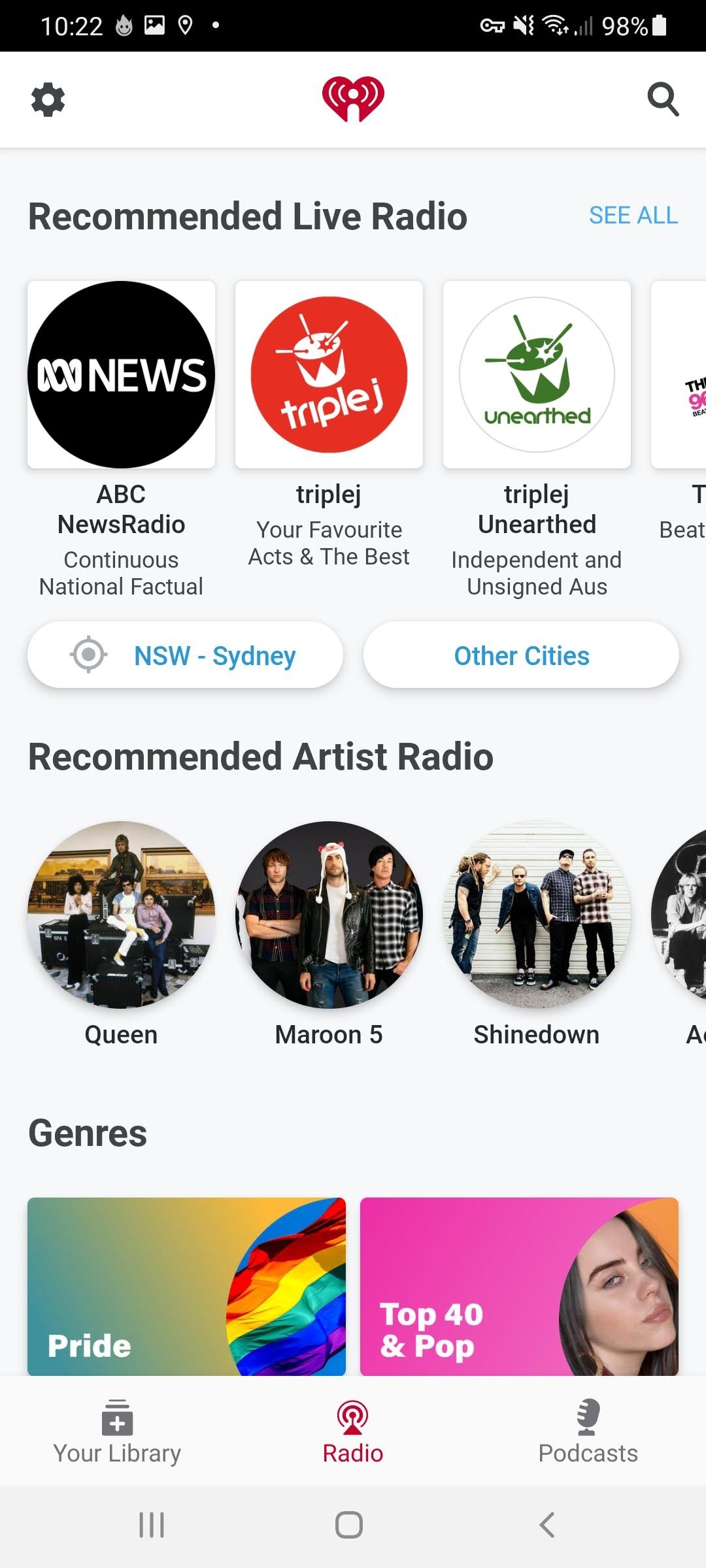This screenshot captures the user interface of the iHeartRadio application. At the center of the screen, there's the iHeartRadio logo: a heart shape with an eye embedded in the middle, emitting sound waves. Navigation icons flank the logo, with a gear icon for settings on the left and a magnifying glass for search on the right, connected by a thin line. Below these icons, there is a heading that says "Recommended Live Radio," accompanied by a blue text button on the right that reads "See All." 

Under this section, thumbnail images represent various radio stations. The first thumbnail is labeled "ABC News Radio" and includes the description "Continuous National Factual." Another thumbnail displays a drum with the Triple J logo and the text "Triple J, your favorite accent, the best..." A similar green drum logo next to it represents "Triple J Unearthed," highlighting "Independent and unsigned Australian bands." The thumbnails can be scrolled horizontally to reveal additional content, but part of a radio icon to the right is cropped out of view.

Further down, two buttons provide geographic radio options: one labeled "NSW Sydney" for New South Wales and another for selecting other cities. The "Recommended Artist Radio" section follows, showcasing artist names and photos within circular frames. Identifiable artists include Queen, Maroon 5, and Shinedown, though one name is difficult to discern.

The "Genres" section below this suggests musical categories with visually distinct icons. The left icon reads "Pride" and features a rainbow flag inset against a gradient background. The right icon says "Top 40 & Pop" on a pink background, with a female singer’s image inset, though her name is not recalled.

At the bottom of the interface are options for accessing "Your Library," "Radio," and "Podcasts," accompanied by a straightforward navigation menu.